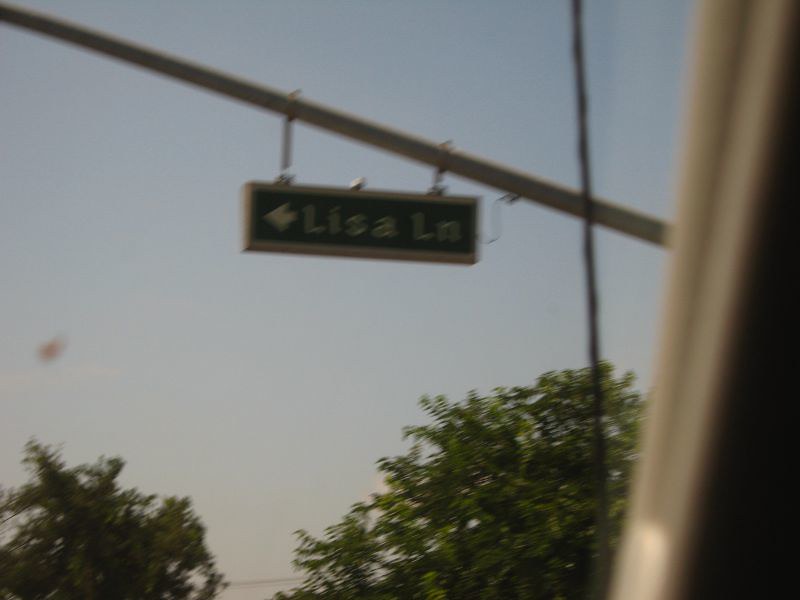A photo captured from the inside of a car, slightly out of focus, showcases an upward view into a hazy, smog-tainted blue sky. Dominating the scene is a horizontal pole from which a street sign dangles, reading "Lease Away." Below the sign and pole, the tops of two trees peek into the frame, adding a touch of nature to the urban setting. The edge of the car's window is faintly visible, grounding the perspective of the photograph as a candid snapshot from within the vehicle.